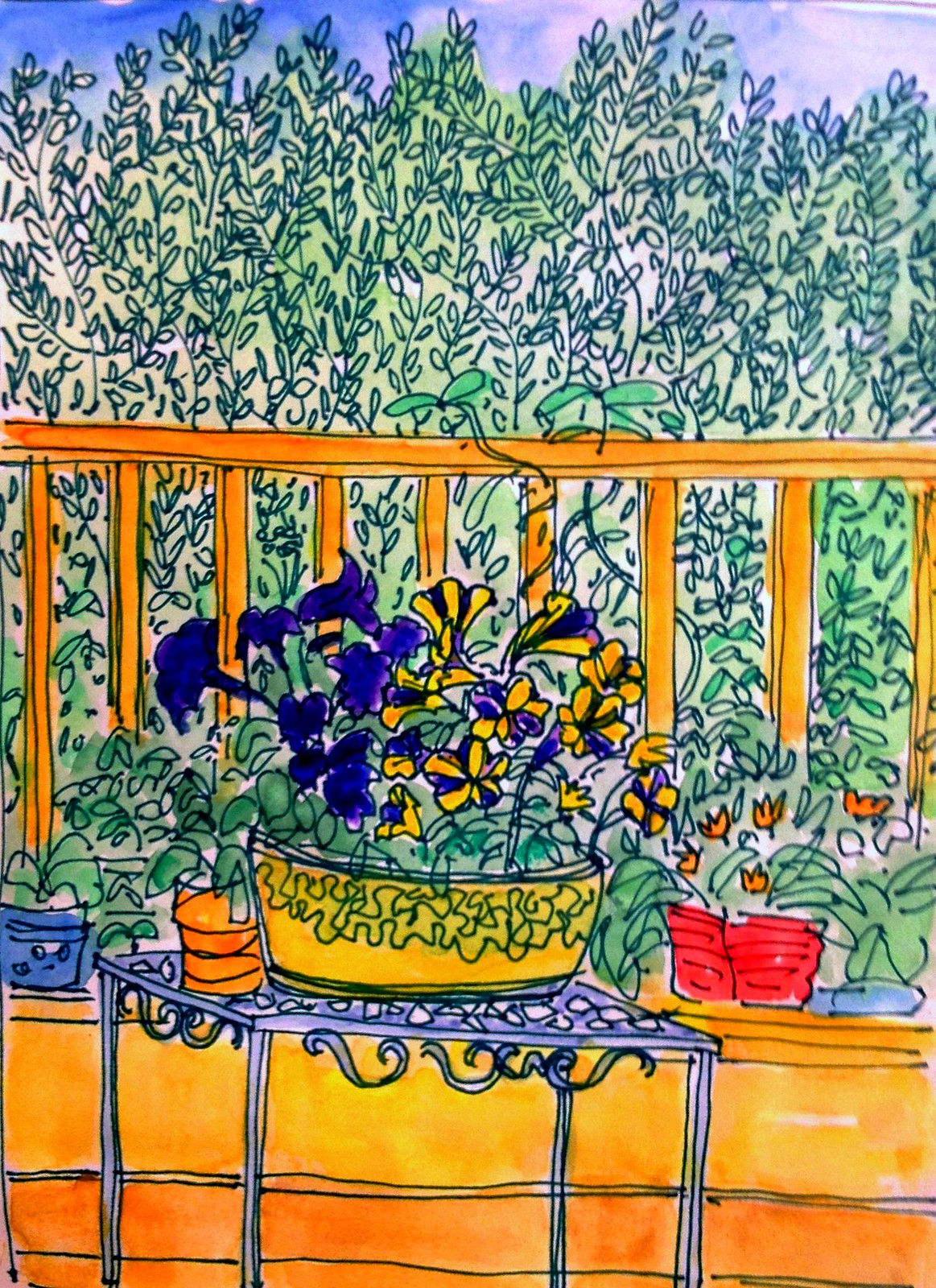This artwork, a vibrant combination of watercolor and ink, depicts a delightful scene featuring a wrought iron table on a brown wooden deck. Centered on the table is a broad yellow pot adorned with squiggly lines, brimming with colorful pansies—purple on the left and a mix of yellow and purple on the right. Beside it, there’s a terracotta pot containing lush greenery. The deck is bordered by wooden railings, entwined with green vines that also cascade down into the background. Additional plants rest against the base of the railing. Above the scene, light green treetops and shrubbery can be seen against a backdrop of a softly brushed blue sky, contributing to the serene, outdoor atmosphere. The image composition hints at an adult coloring book page, thoughtfully brought to life with watercolor accents.